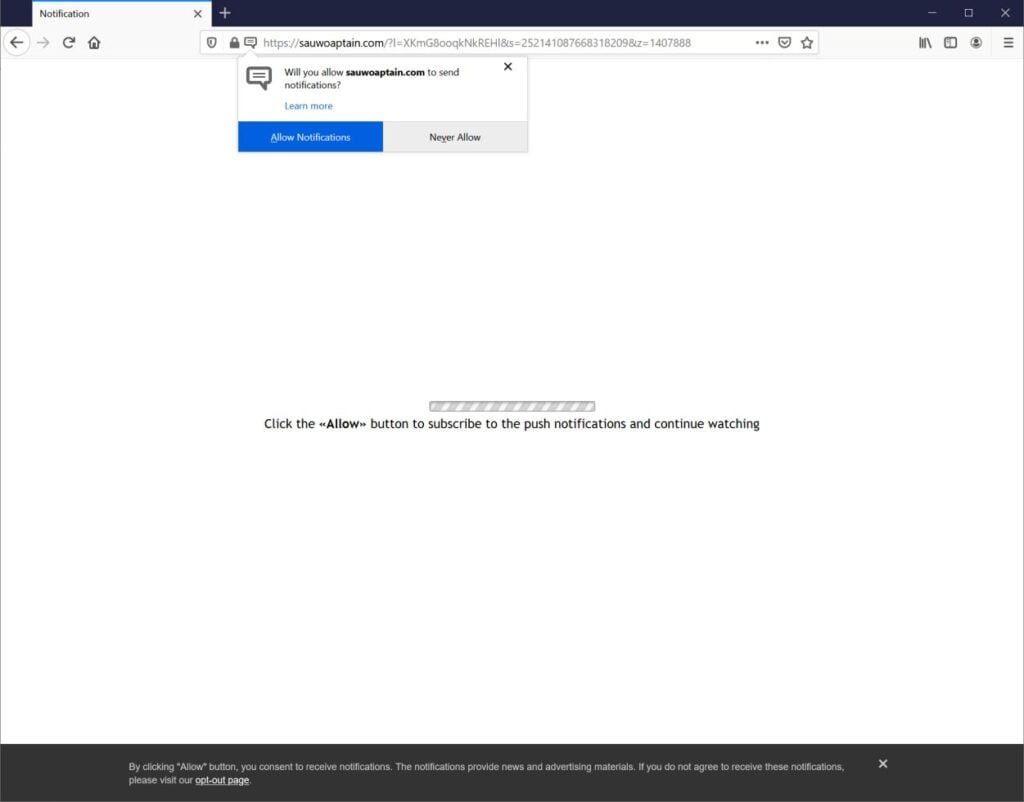The image shows a user interface prompt for allowing notifications. The background is predominantly blue, framed with a black border. At the top, there's a black bar featuring a circular left-pointing arrow, a right-pointing arrow, a refresh icon, and a home icon. Below this bar, a web address is displayed: "sowalkton.com." To the right, there are icons indicating Wi-Fi signal strength, battery life, and user profile.

Beneath this, a gray box contains the main prompt: "Will you allow to send notifications?" The user is presented with two options in blue buttons: "Allow" and "Never Allow." A directive below advises, "Click the arrow button to subscribe to the push notifications and continue watching."